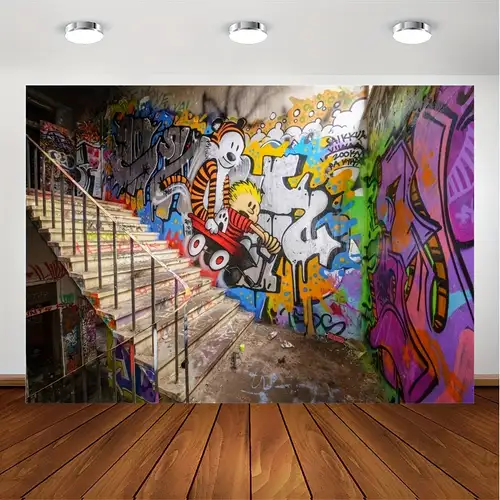The image depicts an interior space that appears to be either part of a home or possibly a museum's urban exhibit. The room features brown hardwood floors with clearly visible wooden planks extending vertically. The ceiling, painted the same light blue as the walls, is fitted with three circular lights. Dominating the scene is a large, wall-height photograph of a stairwell, resembling either a digitally edited photo or a painting of an urban street. The stairs, which are wide and about 12 steps high, ascend to the right, flanked by a wall on the right and a handrail on the left. The walls surrounding the staircase are covered in vibrant graffiti, including a notable image of Calvin and Hobbes riding a red wagon. The graffiti displays a palette of bright colors—purple, green, blue, orange, pink, and white—creating an eclectic and colorful backdrop. The space and artwork together give an otherworldly, almost surreal impression, blending realistic elements with artistic flair.